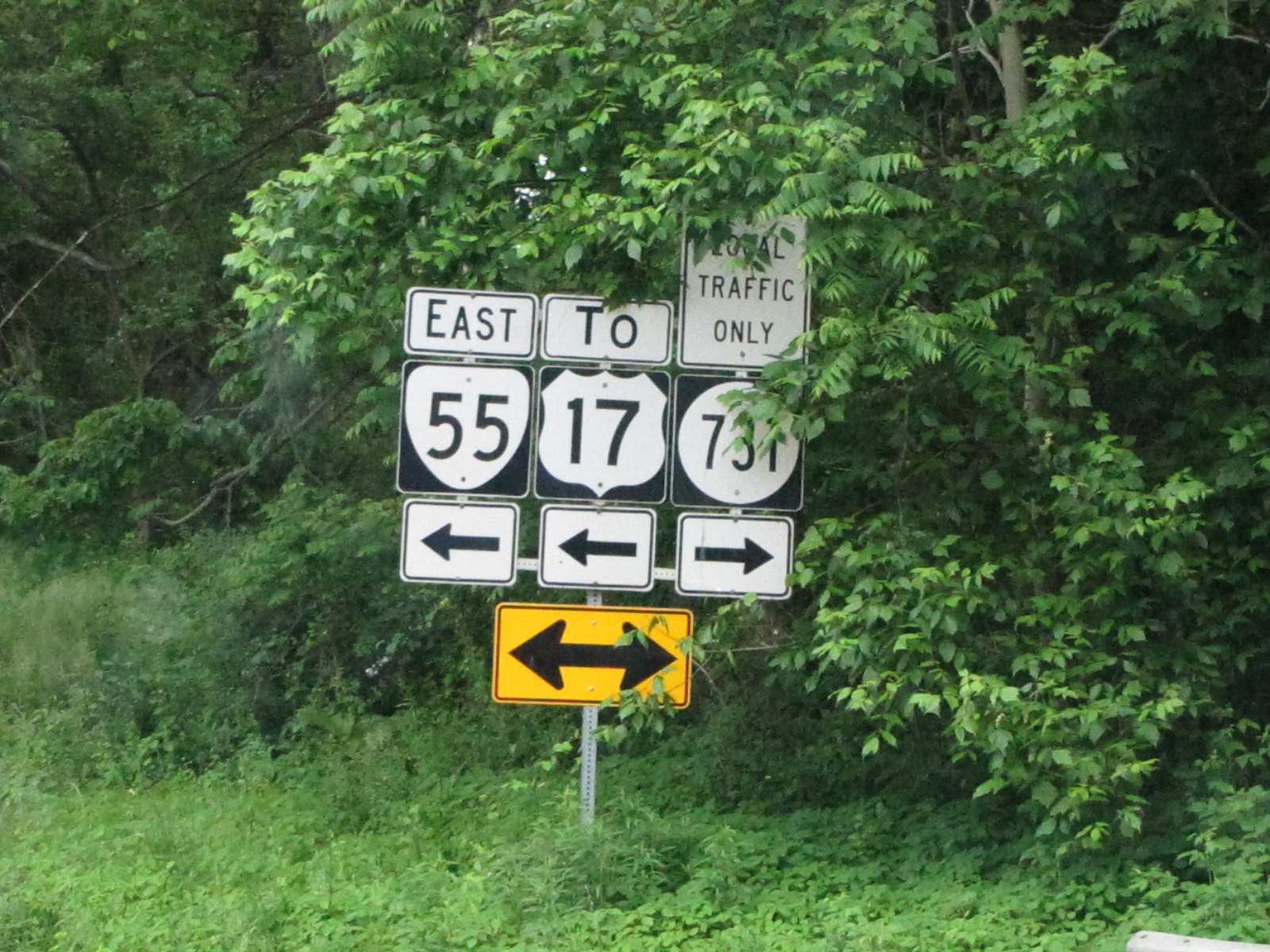This carefully detailed photograph captures a cluster of street signs affixed to a single silver mounting post, set against a backdrop of lush green trees and shrubbery. The scene is framed by nature, indicating that the signs are located on a local road rather than a major highway. At the top left, a white rectangular sign with black text reads "East," accompanied below by a distinctive black-on-white shield-shaped sign for Route 55, with a black arrow pointing left. Adjacent to this, a similar sign designates Route 17 in another unique shield shape, also pointing left. To the right, a square white sign with black text states "Local Traffic Only," partially obscured by leaves but still legible, and beneath it, a circular sign for Route 731 features a black arrow pointing right. Completing the ensemble, a yellow rectangular sign at the bottom displays a double-ended black arrow, indicating two directional flows. The meticulous arrangement of these signs, coupled with their varied shapes and clear directional arrows, provides crucial guidance for local traffic amidst the verdant setting.